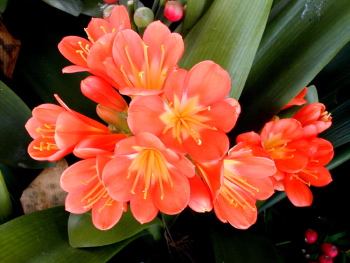This is a detailed close-up, top-down photograph of a cluster of vibrant peachy-pink flowers with orange-yellow centers. The flowers, resembling lilies but also reminding one of honeysuckle, have six or seven petals each and are situated closely together, some with visible stamen-like structures protruding upward. Beneath the blossoms, you can vaguely see green fronds and larger green leaves, with one leaf on the top right appearing darker. The backdrop of the image is predominantly the lush greenery of the plant, but there are noticeable details such as a beige-gray rock and some pink fruit or buds yet to bloom on the bottom part of the image. The photograph is very crisp and emphasizes the contrast between the vibrant flowers and the dark background, making the flowers appear even more vivid.